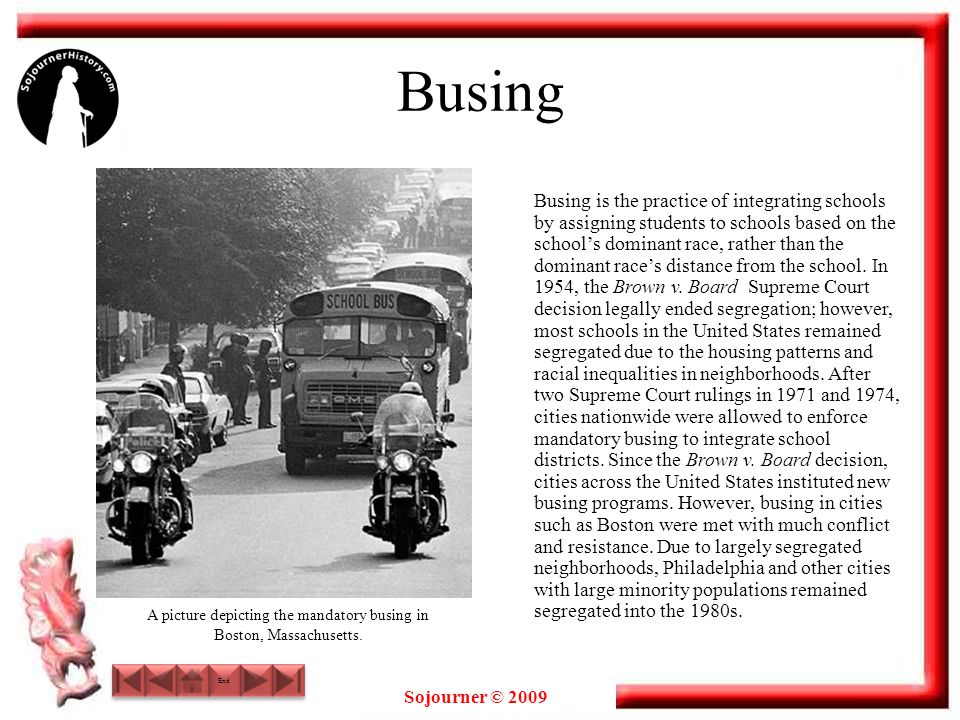A red-framed article showcases a black-and-white photograph in the top left corner, prominently featuring a black circle logo with white text reading "SojournerHistory.com." The bold heading "Bussing" captures attention at the article's top. The image depicts a row of school buses escorted by two police officers on motorcycles, with parked cars lining a tree-filled street. Above the photograph, the caption explains, "A picture depicting the mandatory bussing in Boston, Massachusetts." 

Bussing refers to the practice of integrating schools by assigning students to schools based on the school's predominant race rather than proximity. Despite the 1954 Brown v. Board of Education Supreme Court ruling that legally ended segregation, most U.S. schools remained segregated due to prevailing housing patterns and neighborhood racial inequalities. The text clarifies that following two additional Supreme Court decisions in 1971 and 1974, cities were permitted to enforce mandatory bussing to achieve school district integration. Although many cities, including Boston, initiated bussing programs post these rulings, they faced significant opposition and conflict due to their deeply segregated neighborhoods. Notably, cities like Philadelphia continued to experience school segregation into the 1980s.

At the bottom center of the article, "Sojourner" along with a possible copyright symbol for 2009 is mentioned. To the left, six maroon-colored squares, adorned with sideways triangles on the outer edges and a mysterious pink and white shape, add a unique visual detail. The exact nature of these elements remains unspecified.